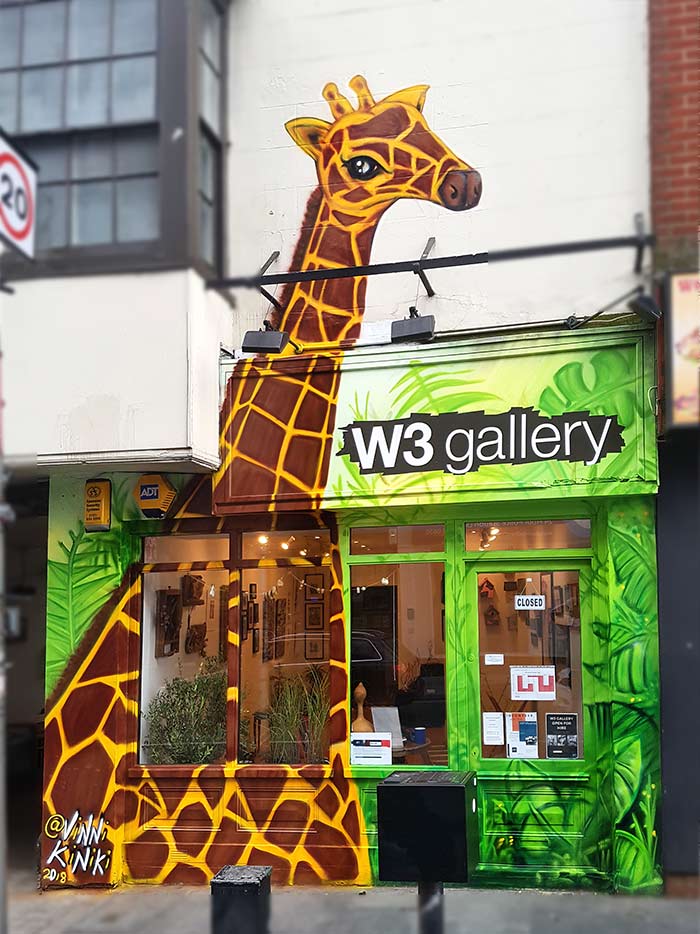The image depicts a vibrant storefront, titled "W3 Gallery," situated in what appears to be a city center. The primary feature of the storefront is an expansive mural of a brown and yellow giraffe, set against lush, green foliage, giving it a jungle-like appearance. The giraffe, painted by artist @Niniki Nikki in 2013, extends to two stories, creating a striking, three-dimensional effect. The facade of the gallery is a mix of detailed greens and a bold, black and white font spelling "W3 Gallery" at the top. The display windows of the gallery are small and rectangular, adorned with plants and various artworks visible inside. A "Closed" sign is prominently displayed on the door, which also bears other notices. The doorway leads into a hallway, suggesting the building extends further back. This thoroughly stylized gallery front, combining natural themes with urban elements, captures the essence of an art-focused retail space.